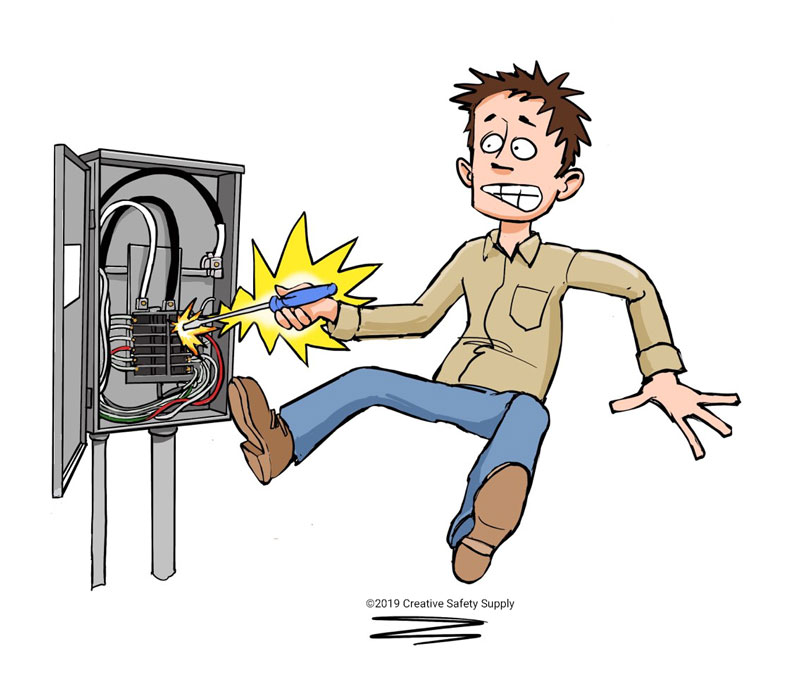In this digital cartoon illustration set against a completely white background, a man with spiky brown hair, wearing a light brown long-sleeved shirt, blue jeans, and brown shoes, is depicted being electrically shocked. His mouth is gritted and his eyes are wide open in surprise, reflecting his grimacing expression as he is jolted into the air. On the left side of the image, his right hand, grasping a blue-handled screwdriver emitting yellow and orange sparks, is inside a gray electrical switchboard. The switchboard, mounted on two gray poles, is an open box containing an array of black switches connected by white, black, red, and green wires. Below the illustration, in small black text underlined, it reads “Copyright 2019 Creative Safety Supply.”